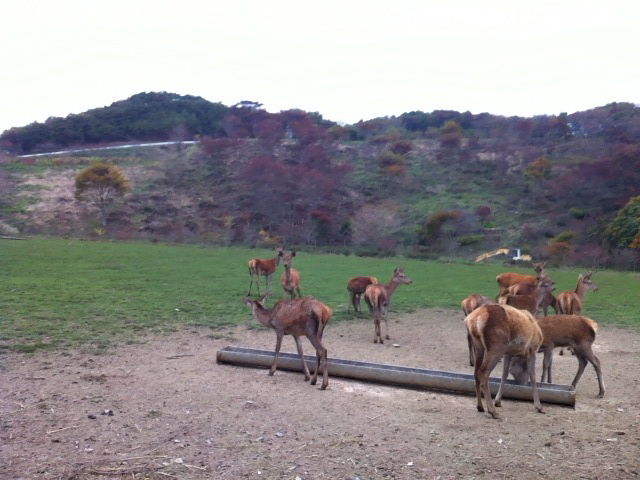The overexposed color photograph, taken outdoors during daylight, captures a pastoral scene with undulating hills in the background. The sky above these hills is virtually white, devoid of any detail due to overexposure. The hills themselves display a patchwork of colors, including dark green, reddish tones, and patches of yellowish-brown. A notable tree with yellowish-brown leaves stands to the left at the base of the hills, while the ridgeline at the top left appears dark green. The hills are adorned with various grasses, trees, and bushes.

In the foreground, the image shows a partially eroded dirt area shaped like a partial rectangle, surrounded by lush, dark green grass. This grassy meadow stretches into the distance, meeting rolling hills lined with trees that have orange, red, and green leaves. A notable feature in the foreground is a metal U-shaped trough, possibly holding water or feed, with a couple of animals, presumably donkeys or deer, drinking from it. 

Approximately ten tan-colored, skinny animals with short fur and no visible antlers are scattered around the trough. Their exact species is somewhat unclear due to the image being slightly blurred and grainy, especially visible across the background foliage and hills. Some animals face the camera, while others look in different directions or are grouped together towards the right side of the image. The photograph also faintly shows a yellow tractor or backhoe in the distant field, adding to the rural ambiance.